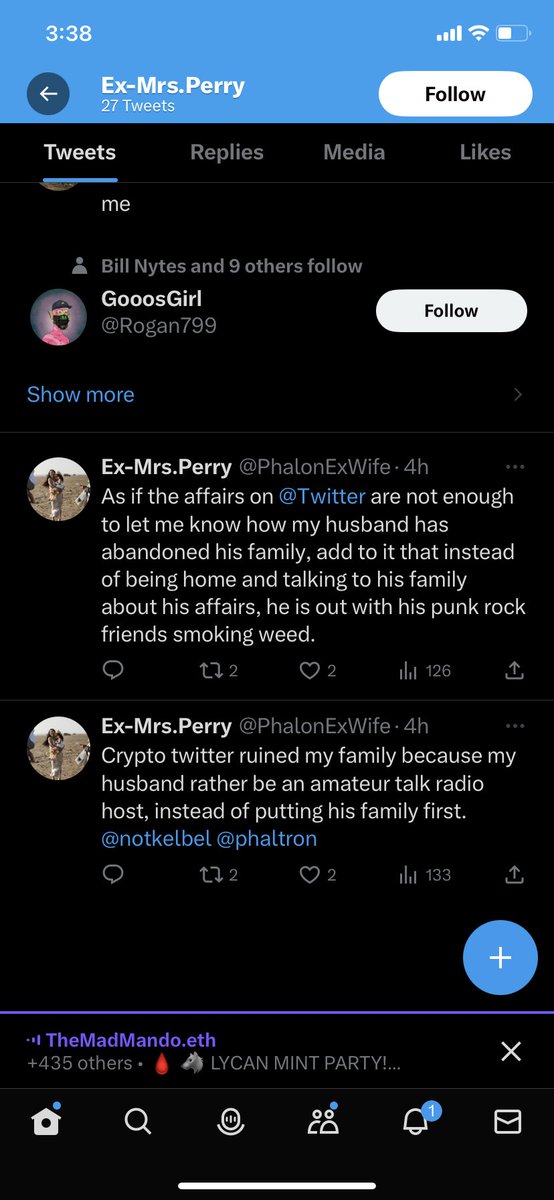In the upper left-hand corner of the image, the time is displayed in white font as "3:38." The title of the visible Twitter account reads "X Mrs. Perry," indicating the user has posted 27 tweets. In the upper right-hand corner, there are several cell phone icons displaying personal signal strength, Wi-Fi connectivity, internet connection status, and battery level.

The screen shows the Twitter interface, suggesting it is an older version before the platform's rebranding to "X." The display indicates that the user "Goose Girl" (@rogan799) is being followed by Bill Nights (NYTES) and nine others. The interface also provides an option to "Show more" tweets.

Two tweets from the user "X Mrs. Perry" are prominent. The first tweet expresses frustration: "As if the affairs on Twitter are not enough to let me know how my husband has abandoned his family. Add to it that instead of being home and talking to his family about his affairs, he is out with his punk rock friends smoking weed." The second tweet from the same user laments: "Crypto Twitter ruined my family because my husband would rather be an amateur talk radio host instead of putting his family first."

Overall, the image captures a glimpse into how social media users often share personal grievances and issues publicly for their followers and the broader internet audience to see.